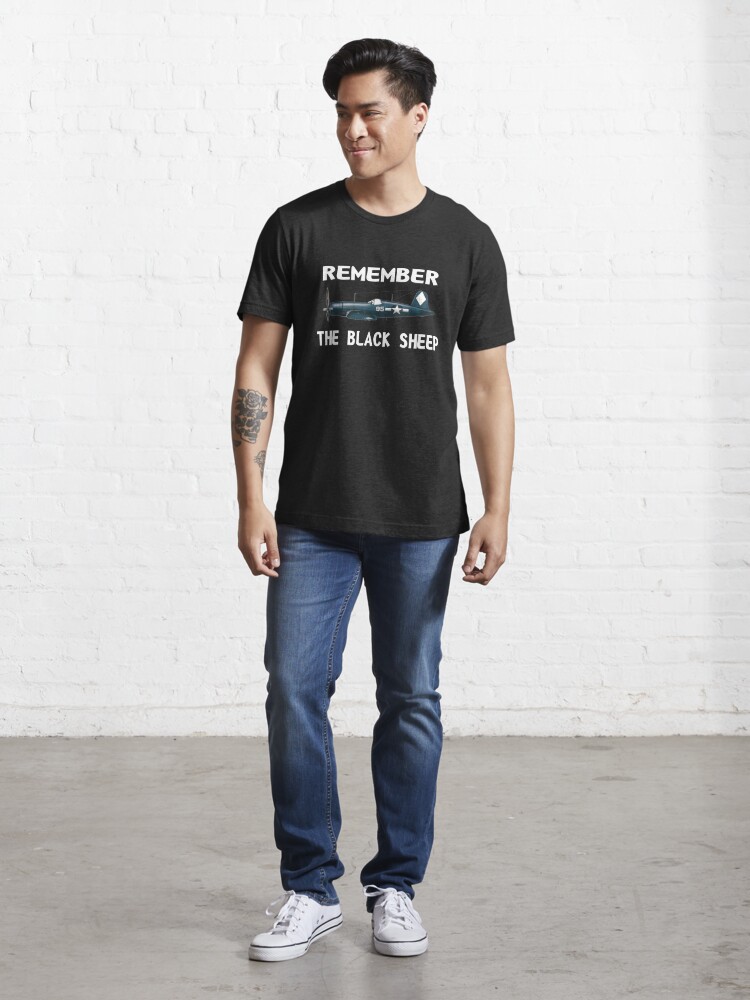In this professionally taken photograph, an Asian man with tan skin and short jet black hair stands smiling and looking to the side. He wears a black t-shirt that features white text reading "Remember the Black Sheep?" along with an image that appears to be a blue submarine or another transportational vessel. His attire is completed with blue denim jeans and white sneakers. Notably, he has a tattoo on his right arm, though the details are hard to make out. The scene is well-lit and focused, set against a white-painted brick background and a gray floor. Despite the clarity of the image, the intent or subject of the advertisement remains unclear as no additional context is provided beyond his clothing and appearance.